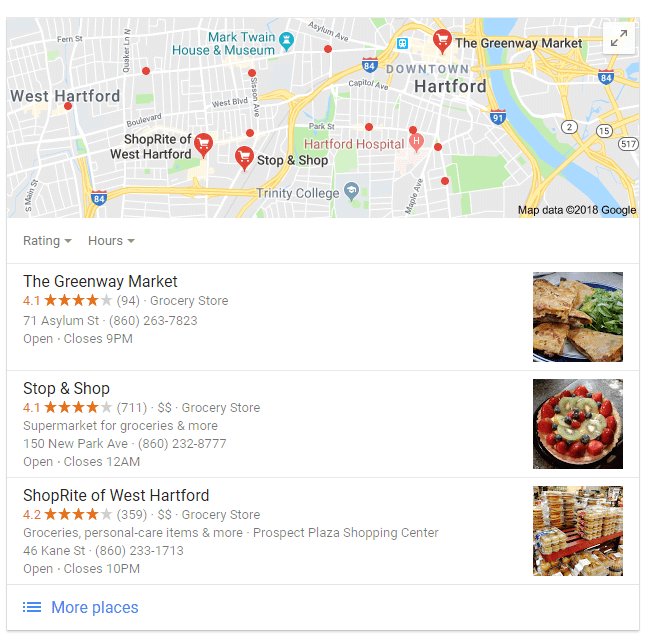In this image of Google Maps search results for grocery stores in the West Hartford area, three highlighted locations are prominently featured: Greenway Market, Stop & Shop, and ShopRite of West Hartford.

1. **Greenway Market**
   - **Rating**: 4.1 stars out of 5 (94 reviews)
   - **Category**: Grocery store
   - **Address**: 71 Asylum Street, Hartford, CT
   - **Phone**: 860-263-7823
   - **Hours**: Currently open, closes at 9 PM
   - **Preview**: Includes a photograph of one of their dishes

2. **Stop & Shop**
   - **Rating**: 4.1 stars out of 5 (711 reviews)
   - **Category**: Grocery store and supermarket for groceries and more
   - **Address**: 150 New Park Avenue, West Hartford, CT
   - **Phone**: 860-232-8777
   - **Hours**: Currently open, closes at 12 AM
   - **Preview**: Includes a photograph of a dish they offer

3. **ShopRite of West Hartford**
   - **Rating**: 4.3 stars out of 5 (359 reviews)
   - **Category**: Grocery store offering groceries, personal care items, and more
   - **Location**: Prospect Plaza Shopping Center, 46 Kane Street, West Hartford, CT
   - **Phone**: 860-233-1713
   - **Hours**: Currently open, closes at 2 PM
   - **Preview**: Includes a photograph of one of their dishes

At the bottom right, there is an option to explore more places, indicated by a hamburger icon labeled “more places.”